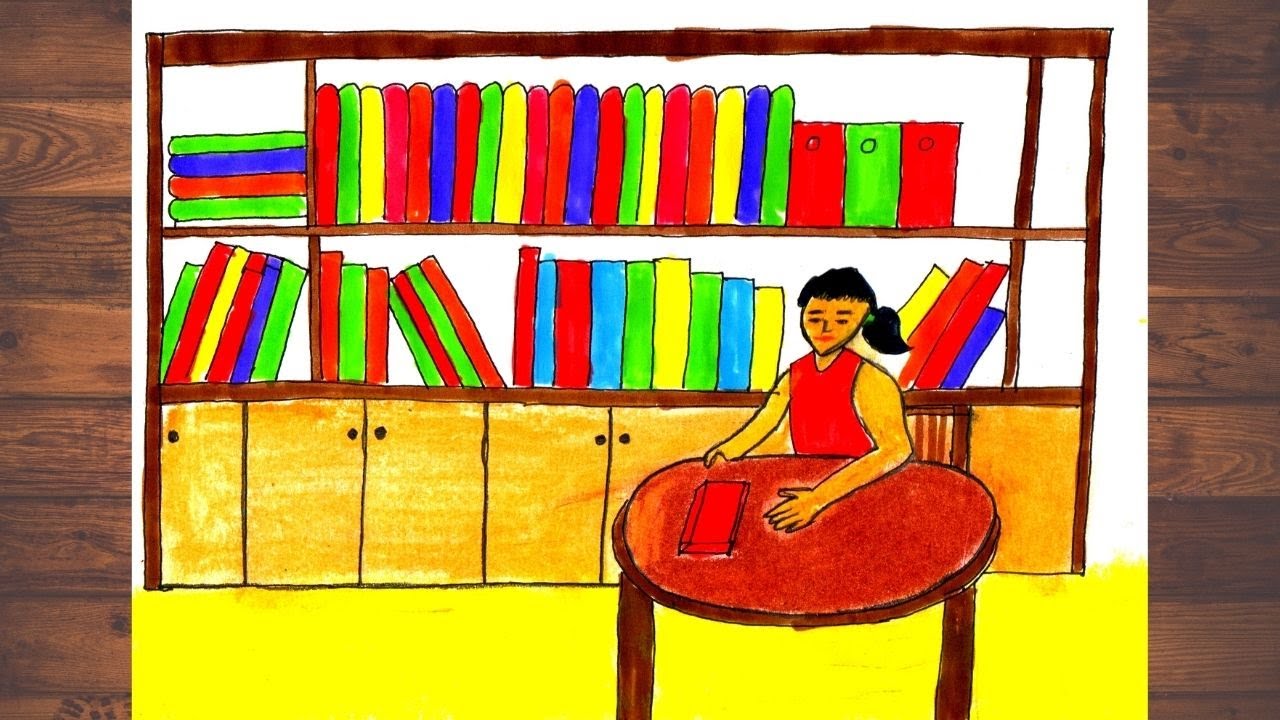This is a vibrant, childlike drawing on an 8.5 by 11-inch white sheet of paper, presumably done by a child aged between 7 and 12 using magic markers. Displayed on a wooden surface, possibly a hardwood floor or desk, the photo of the drawing is taken from directly above. The depicted scene showcases a young girl with yellow skin and black hair tied back, seated at an oval wooden table. She is wearing a red t-shirt and has a red book in front of her on the table, which itself is a darker shade of red. The room features a yellow floor, white walls, and a large dark brown bookshelf with light brown cabinets at the bottom, adorned with knobs. The shelves are filled with variously colored books in shades of red, yellow, blue, green, and light blue.